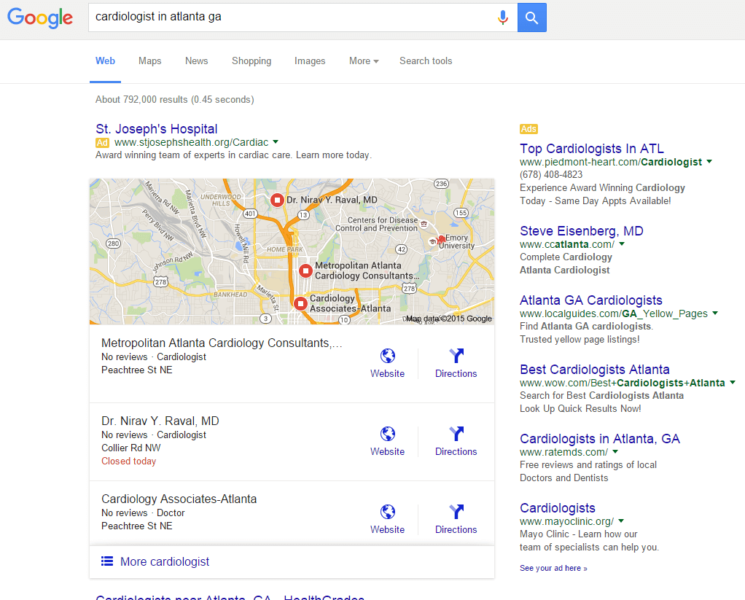The image depicts a Google search results page on a computer screen, with the query "cardiologist in Atlanta, GA" entered in the search bar, highlighted by the multicolored Google logo at the top. To the right of the search bar, there's a microphone icon, and next to it, a clickable search magnifying glass icon.

Below the search bar, there are various navigation options including "Web," "Maps," "News," "Shopping," "Images," "More," and "Search tools." 

The first search result is an advertisement for "St. Joseph's Hospital," highlighting their award-winning team of cardiac care experts, accompanied by a call to action to "Learn more today."

A map follows, displaying three locations marked with red circles containing white squares, indicating cardiology offices. The listed locations include:

1. **Metropolitan Atlanta Cardiology Consultants** - with links to their website and directions.
2. **Dr. Nirav Y. Ravel, MD** - also providing links to the website and directions.
3. **Cardiology Associates Atlanta** - similarly offering website and directions links.

On the right side of the screen, there's an option to click for "more" information, which likely offers additional search results related to cardiologists in Atlanta, GA.